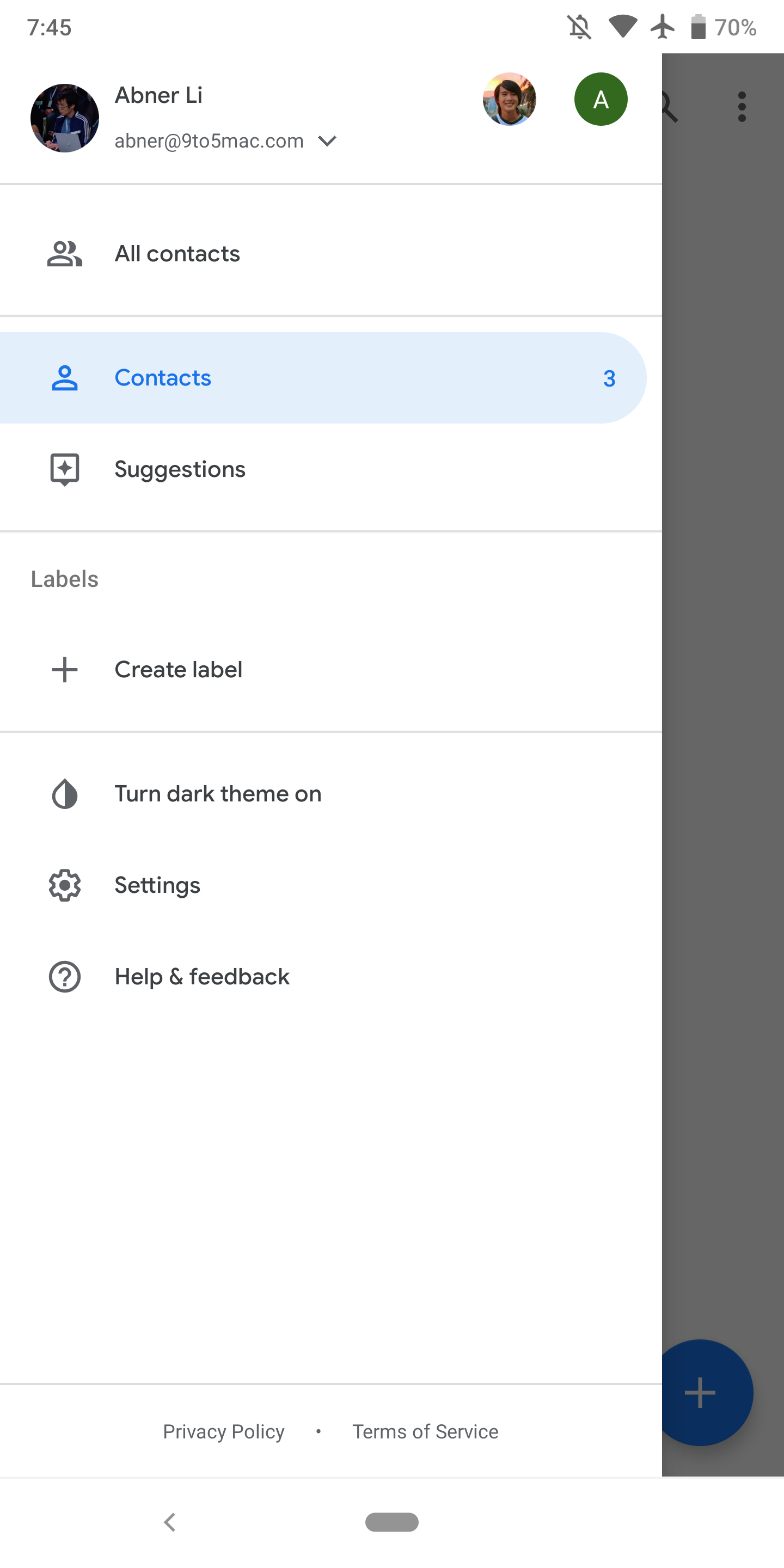This screenshot, captured from an Android phone, displays a detailed view of an app's settings interface. The top bar indicates it is 7:45, with full Wi-Fi connectivity, airplane mode enabled, the ringer set to silent, and the battery at 70% charge. 

The screenshot shows the settings sidebar open. At the top of the sidebar, the username "Amber Abner Lay" is displayed alongside an avatar and a thumbnail image. Amber's email address is also visible beneath her name. To the right, there are two additional avatars: one featuring a face and another with the letter 'A'.

The menu options under the profile information include "All Contacts," "Contacts," and "Suggestions." It also features a section for labels, with an option to "Create Label" accompanied by an add button.

Further down, the menu provides options such as "Turn Dark Theme On," "Settings," and "Help & Feedback." At the bottom of the menu, "Privacy Policy" and "Terms of Service" links are visible, suggesting a comprehensive settings configuration typically found in such applications.